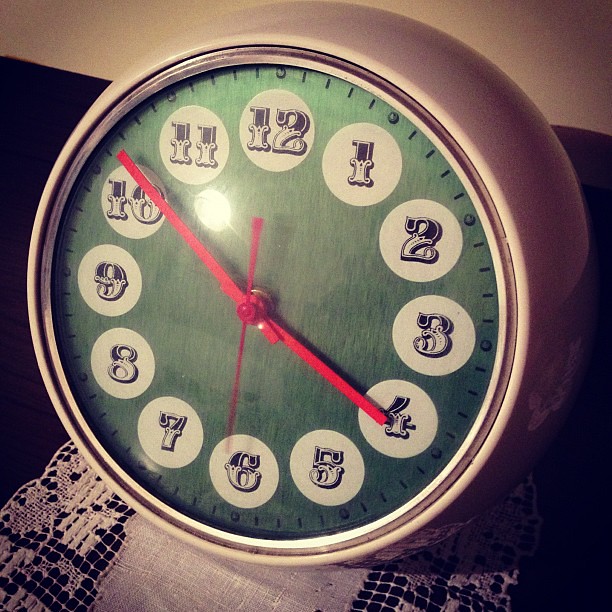This photograph captures a vintage-style alarm clock with a charming, nostalgic appearance. The clock features a round face with a pale green background adorned with ornamental white numerals, reminiscent of circus fonts from the Western period. These numerals are arranged in a traditional circular pattern for easy readability. The clock is distinguished by its vibrant red minute, hour, and second hands, which stand out strikingly against the green backdrop. The exterior of the clock is a sleek white, likely metallic, as indicated by the shine and reflection on its surface. The clock is positioned on what appears to be a cabinet or dresser, with a white cloth placed between the surface and the clock. The setting is dimly lit, and the background wall is white, providing a neutral contrast to the clock's vivid colors.